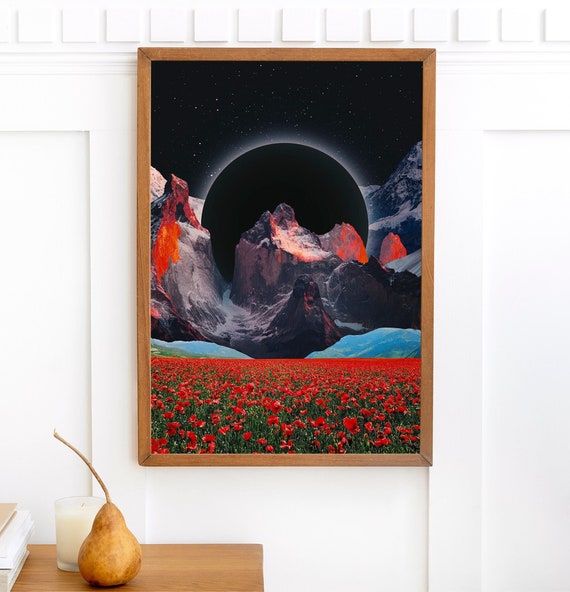The image captures an indoor setting with a vertically aligned, almost square, portrait-style picture frame hung on a textured white wall with white cutout sections. In the lower left corner of the image, there's a small wooden table with visible corner edges, holding an assortment of items: a large potato with a stem, an unlit white candle, a pair of pears, and a stack of books or papers with frosted glass covers. The picture frame itself is medium brown wood, containing a detailed illustration. The top of the picture features a pitch-black, starry sky with tiny white speckles and a black circular moon with a subtle glow around its edges, resembling an eclipse. Below the sky, there's a rugged mountain range with a blend of grays, blacks, whites, and vibrant oranges that give the impression of volcanic activity or lava. At the bottom of the picture, there's a lush green field dotted with an abundance of red flowers, enhancing the vivid and contrasting elements within the frame.